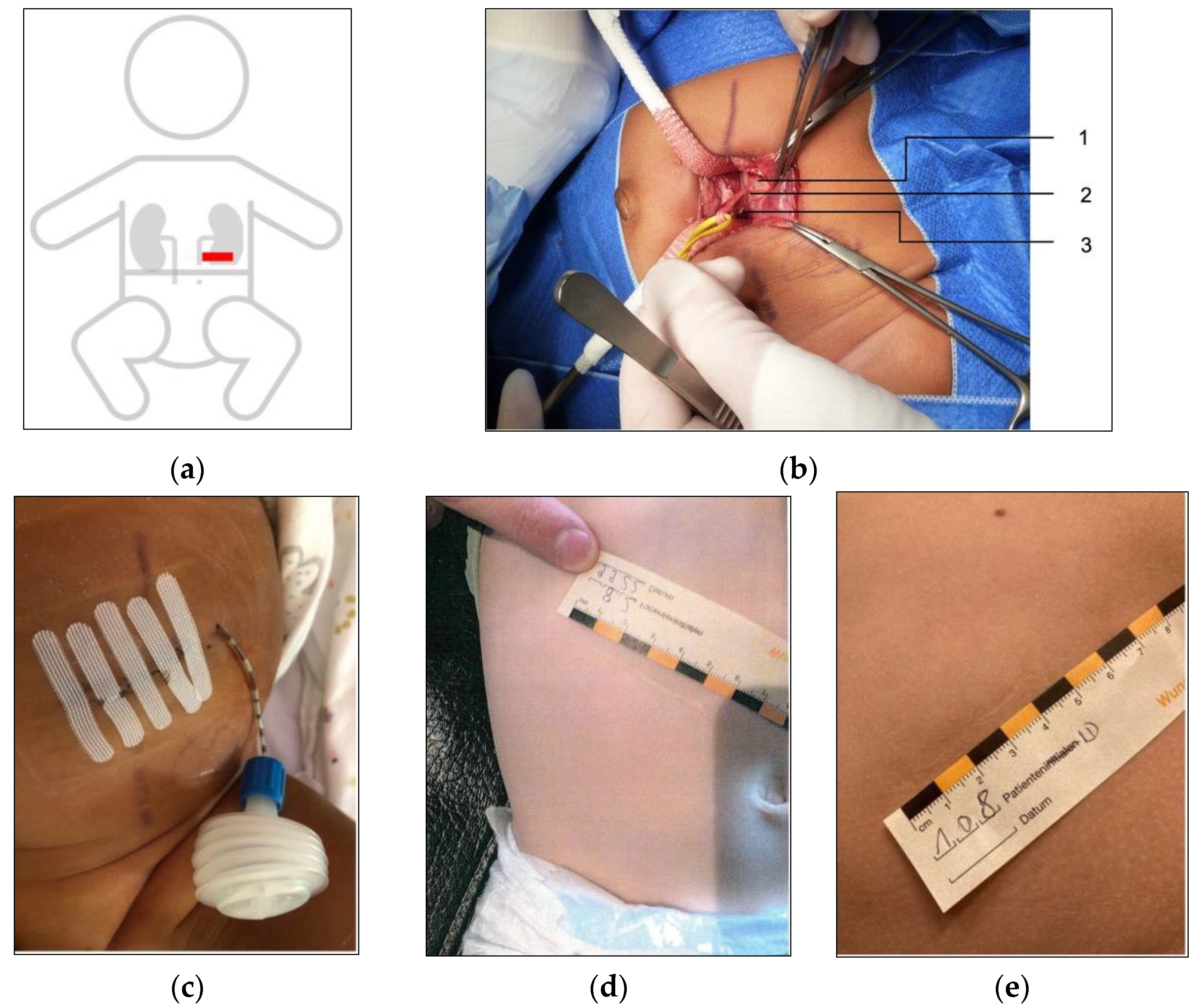This detailed image depicts a step-by-step guide to a surgical procedure on an infant, combining a line art illustration with four color photographs. In the top left corner, labeled (A), is a portrait-oriented line drawing of a child's body with a gray outline and a red vertical stripe indicating the surgery site over the kidneys. To the right, labeled (B), is a color photograph of the surgical operation, showcasing the open wound surrounded by blue drapes and numerous surgical instruments, with key areas numbered 1, 2, and 3. Below these images, the bottom left photograph, labeled (C), displays the closed incision site, now secured with white adhesive tapes and a drain attached to the right side. The middle photograph, labeled (D), shows a ruler placed above the incision for scale. The final image on the bottom right, labeled (E), is a closer view of the area, providing a detailed measurement of the scar with a ruler.